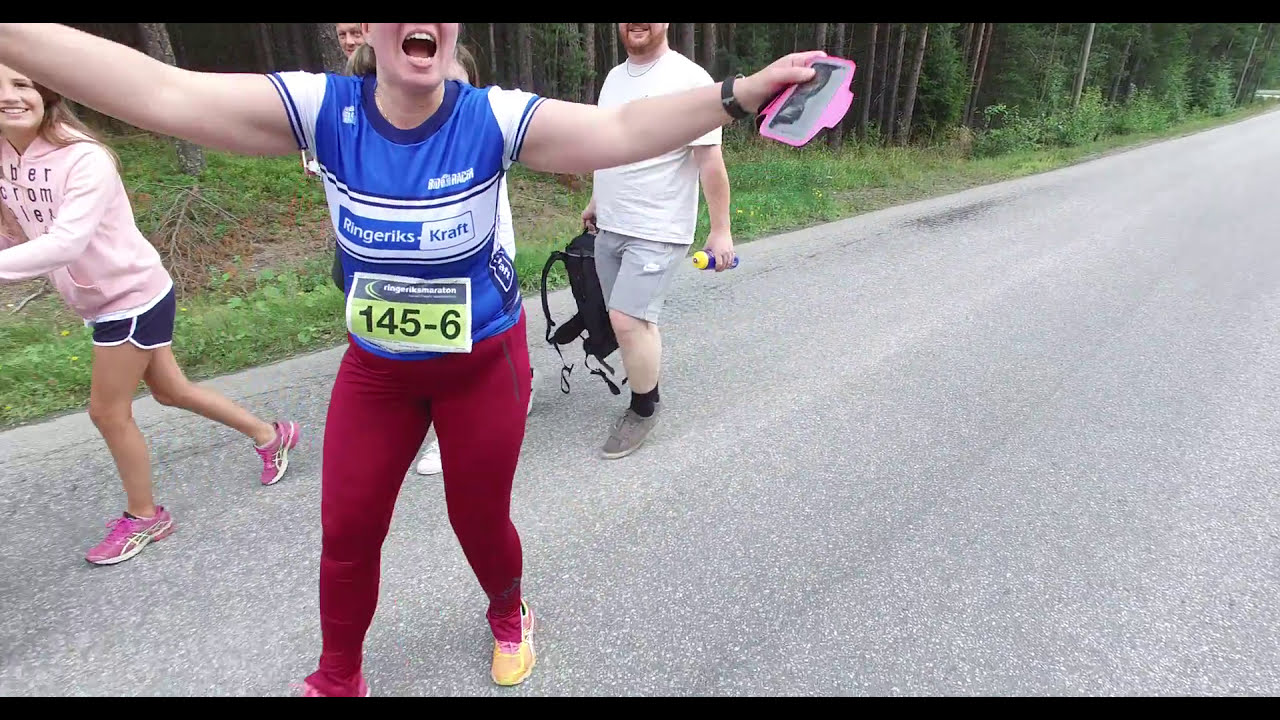The image depicts a lively scene on an asphalt road that stretches diagonally from the bottom left to the top right. The focal point is a woman in the middle left of the frame, seemingly participating in a marathon, as indicated by the pinned paper bearing the number 145-6 on her blue jersey that reads "Ringerisk Craft." She sports red tights and orange shoes. Her blonde hair is somewhat visible, and one of her outstretched arms holds a hot pink protective case, likely for a cell phone. Behind her and slightly to the right is a man smiling broadly, holding a black backpack in his right hand and a blue and yellow-tipped water bottle in his left. He wears gray shoes, black socks, gray shorts, and a white cotton t-shirt, and has a brown handlebar mustache and beard. To the left of the main runner is a young teenage girl, approximately 13-14 years old, dressed in a pink jacket that says "Abercrombie," black shorts with white lining, and dark pink shoes. She has brown hair and is smiling towards the camera. The background features a dense forest of green trees, lending a natural ambiance to the setting. The overall atmosphere suggests an organized outdoor event captured in mid-motion.